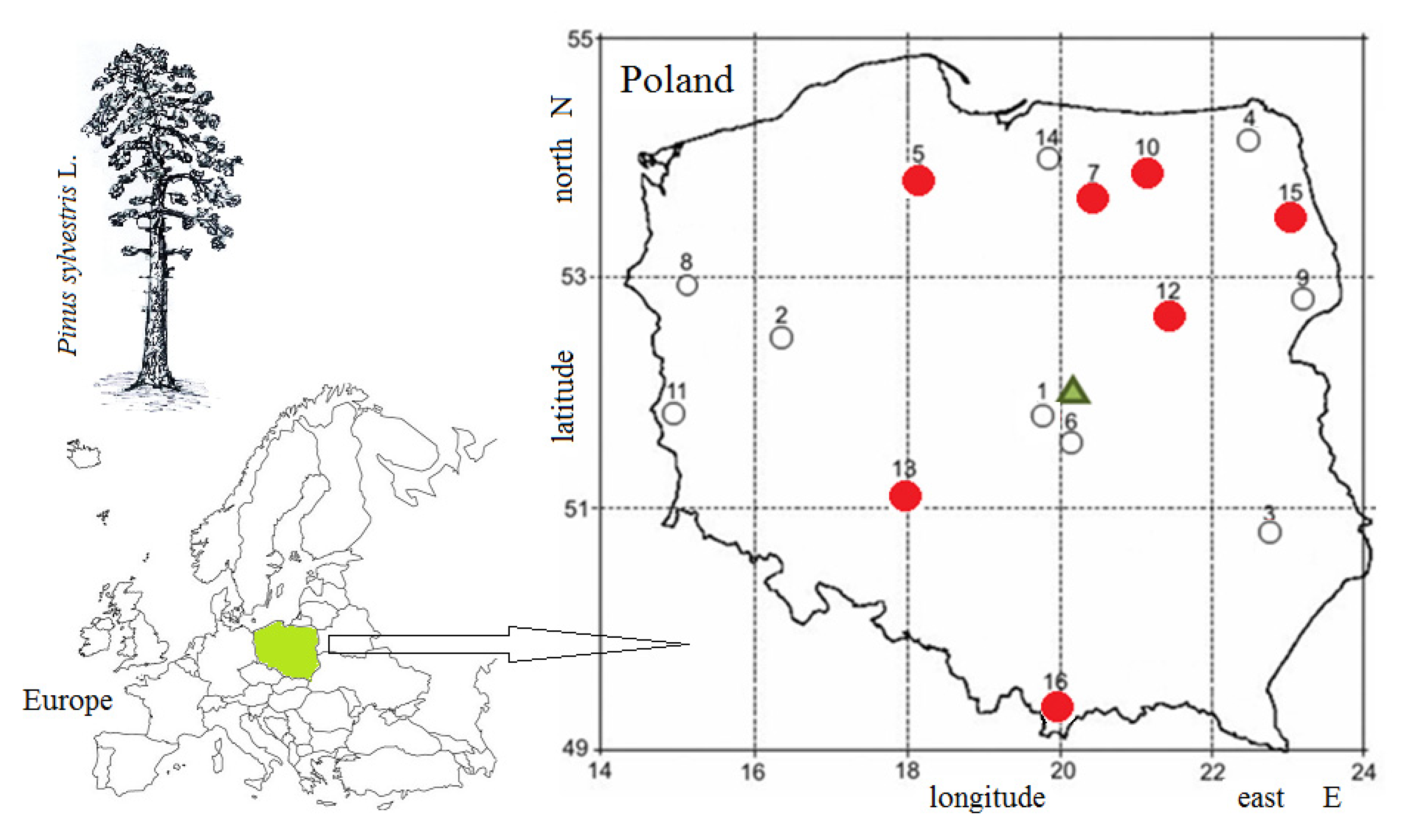The image is a detailed diagram consisting of multiple elements on a white background. At the top left, there is a black and white illustration of a tree labeled "Pinus sylvestris L." Below this, there is a simple line map of Europe, where Poland is highlighted in a bright green color. An arrow points from this map to a more detailed map of Poland on the right. This map of Poland is overlaid with a grid showing latitude (49° to 55° North) and longitude (14° to 24° East) coordinates. Throughout the map, various locations are marked with red dots, white circles with black outlines, and a green triangle. The red dots, numbered 5, 7, 10, 15, 12, 18, and 16, are primarily concentrated in the northern and eastern regions, with a couple in the south. The white circles, numbered 1 through 14, are scattered across the country, avoiding the extreme southern region. The green triangle is slightly off-center, possibly indicating a significant location. The bottom left of the image contains another smaller map of Europe, further contextualizing Poland's location on the continent.